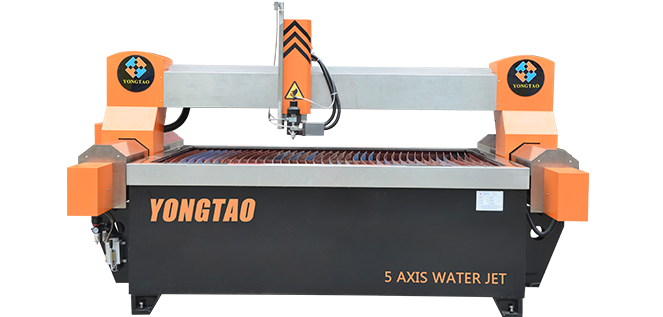The image depicts a sophisticated piece of machinery against a white background, identified as a "Yongtai" branded 5-axis water jet cutter. The machine features a predominantly black base set on plastic legs, topped with a silver grate. The machine's periphery includes orange and stainless steel elements that extend across both ends and form an arm that arches over the top, decorated with the logo "Yongtai" and the label "5-axis water jet" in orange letters at the bottom.

This arm, which has a significant metal rod, appears to house intricate components and wires, suggesting its capability to move horizontally to perform its operations. The arm and rod mechanism looks suitable for sophisticated manufacturing tasks, potentially involving precise cutting or shaping using water jets. The design also includes a visible motor and a cable on the left side, enhancing its industrial appearance. Despite not having any material currently being processed, the machine's detailed and robust build indicates advanced functionalities in fabrication or engineering applications.